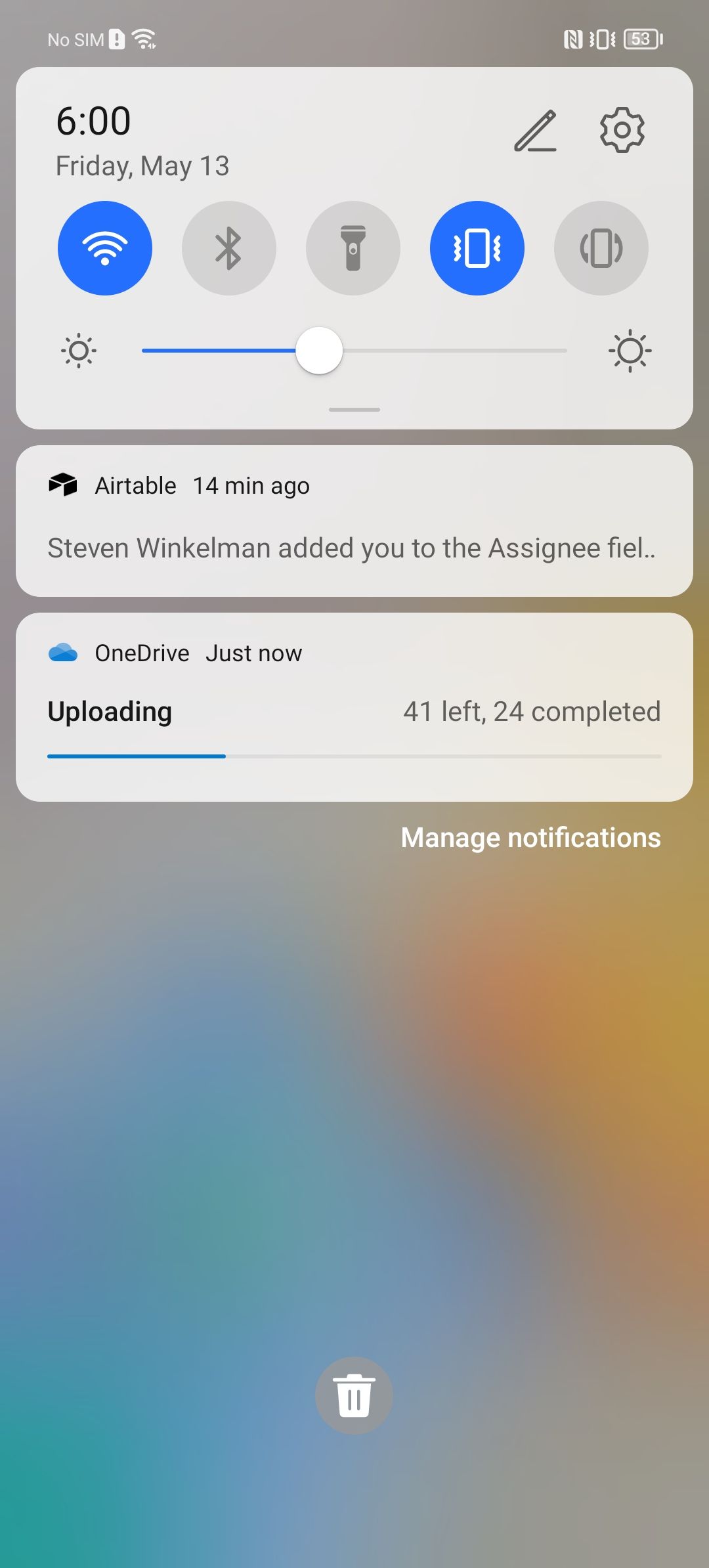The image showcases the notification center of an Android smartphone, pulled down from the top to display recent notifications and quick settings. At the top part of the screen, several shortcut buttons are visible. The Wi-Fi button is enabled and shown in blue, the Bluetooth button is disabled and in grey, the flashlight button is in the center and off, represented by a grey icon. The vibrate mode is active and shown in blue, while the screen rotation lock is off and grey. Above the shortcut buttons, there's a settings icon towards the top right corner and a recognition icon next to it. The current time is displayed on the left side as 6:00, and the date is Friday, May 19.

Beneath these shortcuts, there's a brightness slider with a blue gradient on the left side and grey on the right, the slider wheel positioned near the midpoint indicating medium brightness.

The first notification, written in white, mentions that 14 minutes ago, Steve Winkleman added the user to the "assignee" field in a table or task. The second notification is from OneDrive, just now, indicating that a file upload is in progress. The status shows that out of 65 files, 24 have been completed while 41 are remaining.

Towards the bottom right of the notification center, there is a "Manage notifications" button, and at the bottom, there is a delete button to clear notifications.